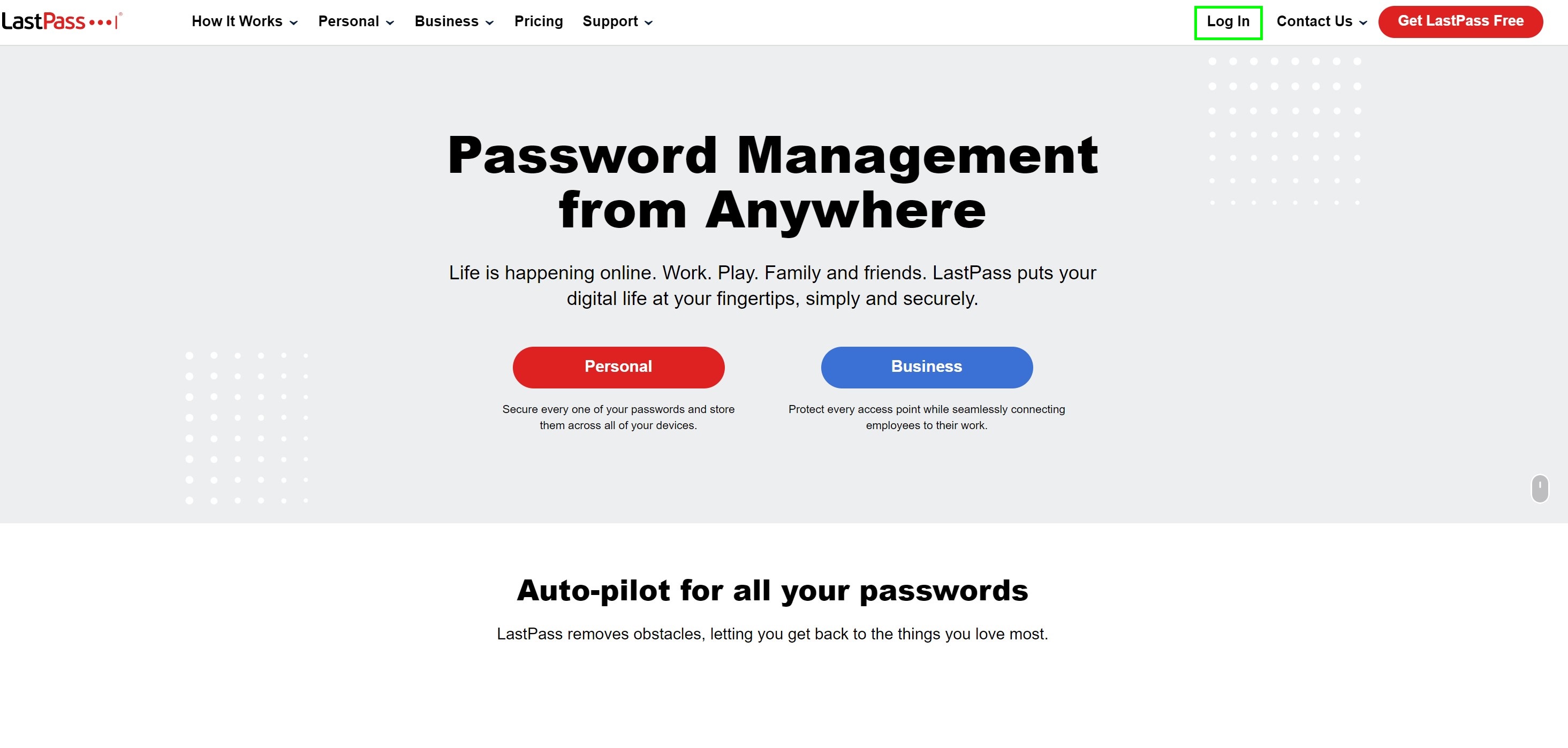Screenshot of the LastPass website:

At the top of the webpage, the LastPass logo is displayed prominently in black and red. Below the logo, there is a series of navigation submenus in black with accompanying arrows, including: "How It Works," "Personal," "Business," "Pricing," and "Support." To the far right of these options is a "Log In" button highlighted by a lime green box, followed by a "Contact Us" drop-down menu. Adjacent to these is a bold red banner with white text that reads, "GET LASTPASS FREE."

Beneath the navigation bar, a large gray box occupies a significant portion of the screen, featuring centered text and buttons. Scattered white dots appear in two clusters as a subtle background element. The main text reads, "Password management from anywhere. Life is happening online. Work, play, family, and friends. LastPass puts your digital life at your fingertips simply and securely." 

Two prominent buttons are positioned below this text: a red button labeled "Personal" and a blue button labeled "Business," each with corresponding black text underneath providing further details on the respective plans.

Further down, a white section announces, "Autopilot for all your passwords," in bold black font. The description below states, "LastPass removes obstacles, letting you get back to the things you love most."

Overall, the screenshot is clear with a readable, decent-sized font, and no pixelation or blurring, ensuring ease of understanding for viewers.